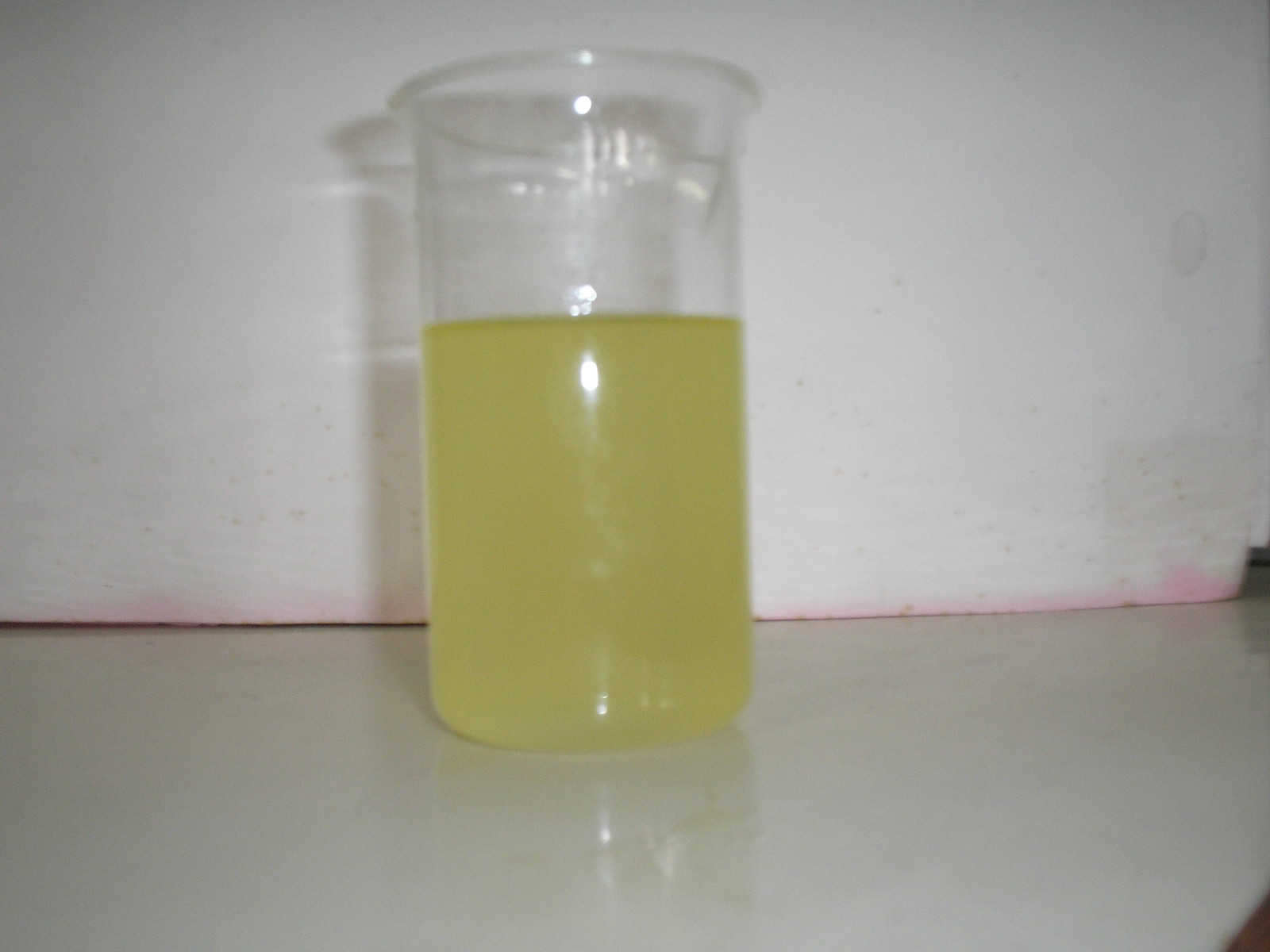The photograph showcases a clear cylindrical beaker, either made of plastic or glass, which stands centrally in the image. It is approximately two-thirds filled with a transparent yellow liquid, the nature of which is unspecified. This beaker is positioned on a white, glossy, reflective surface, potentially a counter or table, which exhibits faint yellow grain, giving it a marble-like appearance. The background features a white material, possibly a piece of styrofoam or a white piece of particle board, with a distinct pink or purple stain along its bottom edge. The lighting in the image creates multiple reflections on both the beaker and the glossy surface, enhancing the clarity and color detail of the yellow liquid inside the beaker.